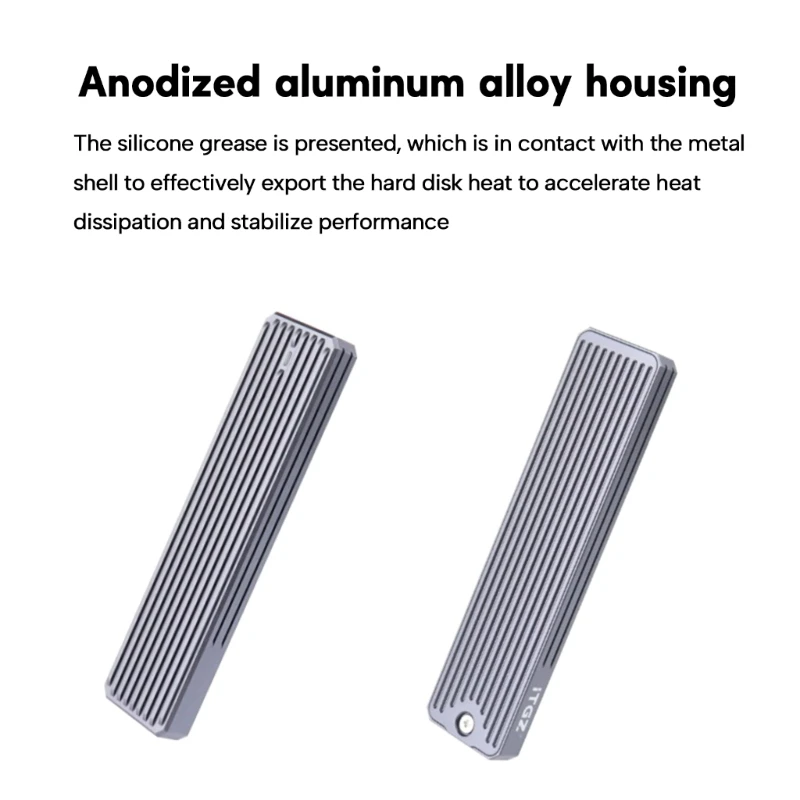The image resembles a professional advertisement set against a white backdrop, showcasing two metallic, rectangular pads that might be aluminum alloy heatsinks. These pads, which feature elongated indented lines running along their length, are marked with the text "ITDZ" or "ITOZ". The pads are positioned side by side, with slight spacing between them, and cast shadows, adding depth to the visual. Above the pads, the text reads: "Anodized aluminum alloy housing. The silicone grease is presented, which is in contact with the metal shell, to effectively export the hard disk heat to accelerate heat dissipation and stabilize performance." The overall scene is meticulously arranged to highlight the functionality and design of the components, likely intended for dissipating heat in electronic devices.